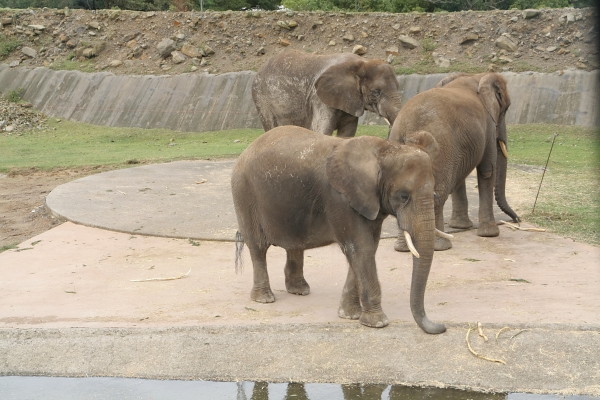This image captures three grey elephants standing on a light grey cement surface, seemingly within a zoo enclosure. In the foreground, there is a small body of water that reflects the nearest elephant. This elephant has large white tusks and an S-shaped trunk that touches the ground. Two elephants stand behind it; one is facing away, only partially visible with its back towards the camera, while the other mirrors the positioned trunk of the first elephant, though further back. All elephants exhibit classic gray skin, with one of the elephants displaying white markings indicative of old age. In the background, there is a cement wall topped with rocks, leading up to a sloped embankment of rocky soil. Beyond this wall, a strip of green grass adds a touch of color to the otherwise earth-toned scene, which includes the dusty ground and the concrete surfaces where the elephants stand.